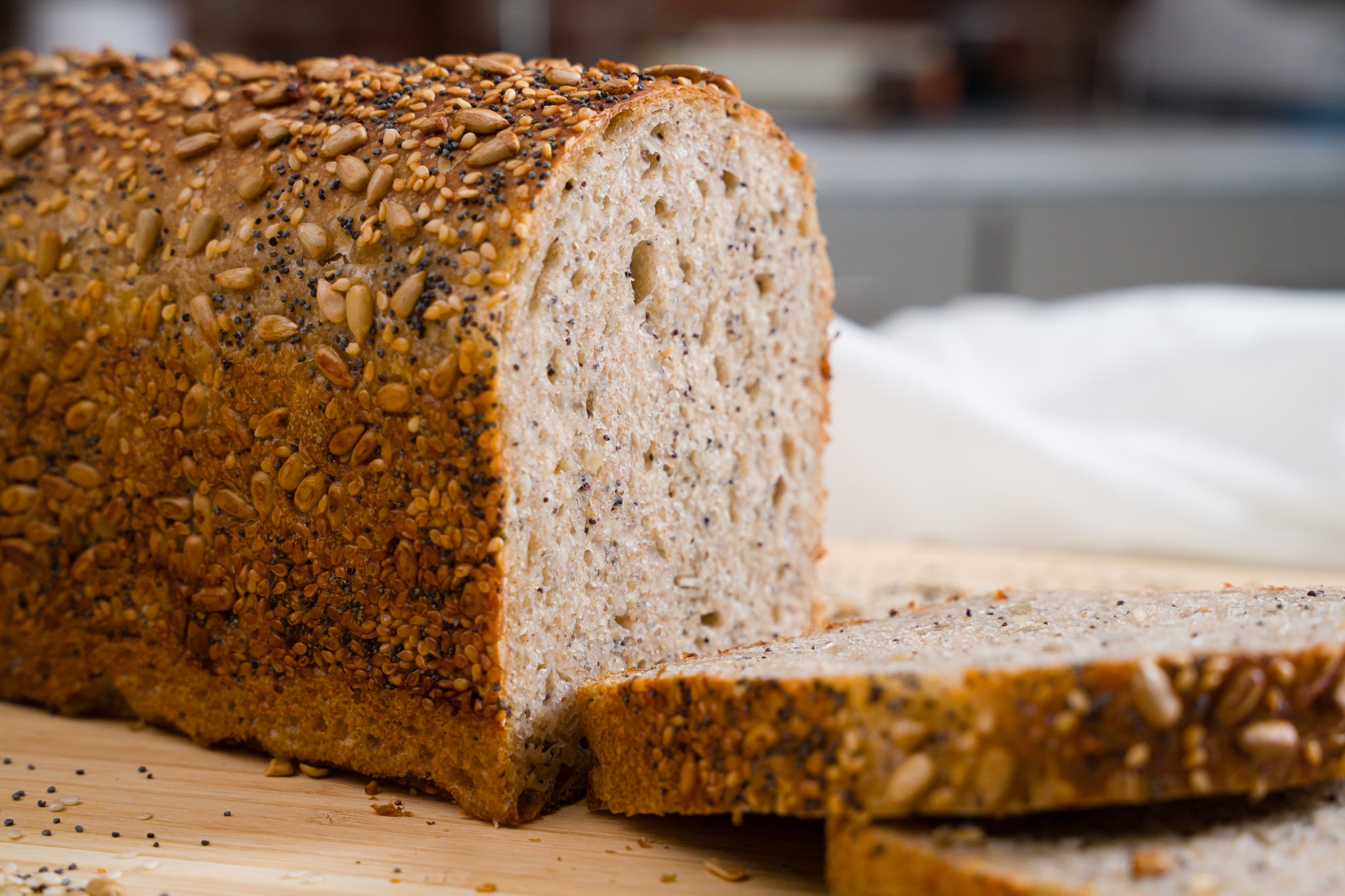This is a close-up photograph of a sliced loaf of multi-grain, nut and seed bread, artistically displayed on a wooden cutting board. The loaf appears to be homemade, with its crust coated in a variety of seeds, including sunflower and possibly poppy seeds. The bread has a wholesome, rustic charm, with a dark brown crust contrasting its lighter, creamy interior, which reveals the nuts and seeds embedded within. Loose seeds are scattered around the cutting board, adding a touch of natural texture. Although the background is blurred, it suggests a kitchen setting with a white tablecloth and a countertop, enhancing the cozy, homely atmosphere of the scene. The image could well be part of an advertisement or social media post showcasing this healthy, delicious-looking artisan bread, ready for making a nutritious sandwich.